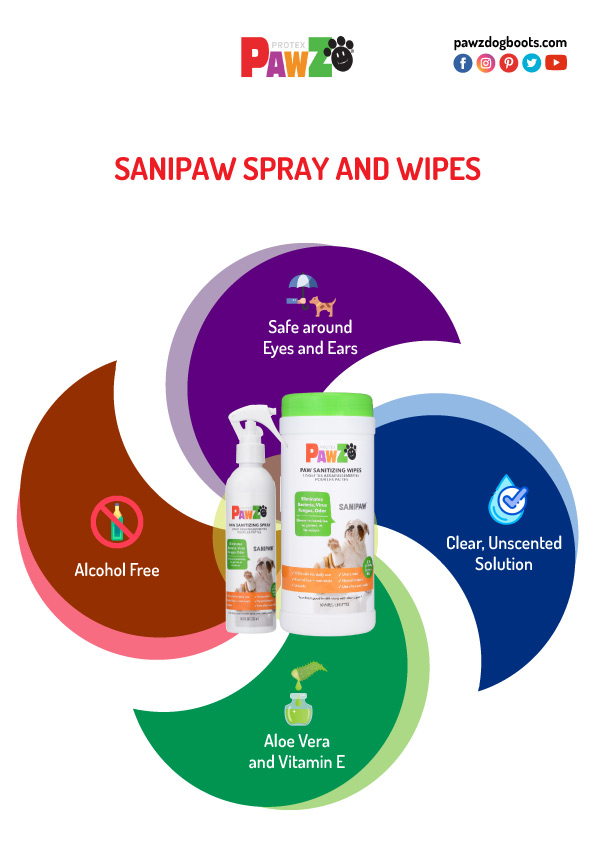The image is a vibrant product advertisement for PAWS, featuring bold, colorful branding elements and detailed product information. The brand name, PAWS, is prominently displayed at the top with a large bold red P, a smaller purple A and yellow W, and a large bold Z. In tiny letters between the P and Z, the word "Protex" is visible. Adjacent to the brand name is an image of a black dog paw print. In the top right corner, the URL "pawsdogboots.com" is displayed.

Below the brand name, the image promotes Sanipo Spray and Wipes, featuring a clear depiction of the products. The spray bottle has a white background and shows an image of a dog with the PAWS branding. The container of wipes also has a white background, an image of a dog, the PAWS branding on top, and a green lid. Surrounding the product images is a circular pattern with multi-colored segments highlighting key features: "Alcohol-Free," "Aloe Vera and Vitamin E," "Clear Unscented Solution," and "Safe Around Eyes and Ears." This advertisement meticulously combines color, text, and imagery to convey detailed information about the PAWS products and their benefits.